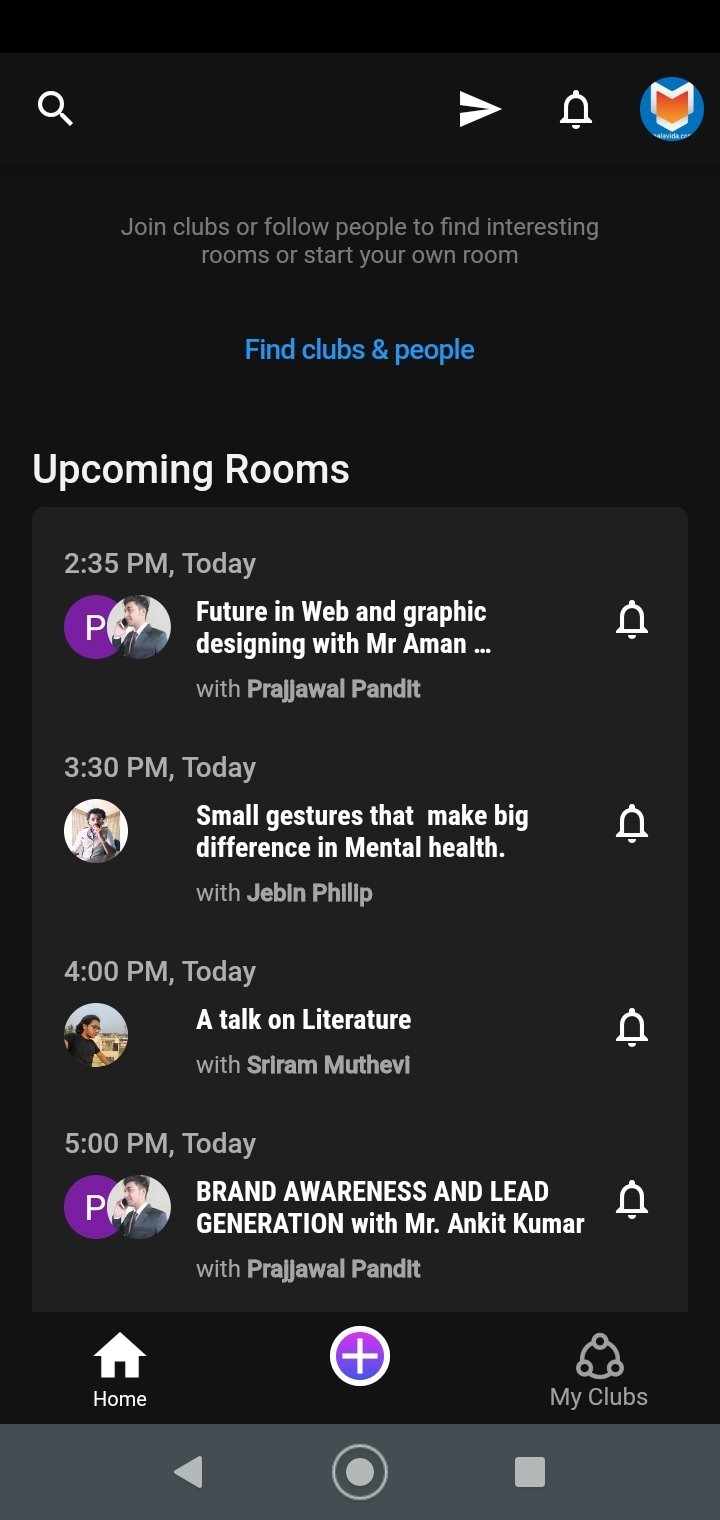The image features a solid black background and appears to be a screenshot from a cell phone displaying a social media post. In the center of the image, there is light gray text that reads, "Join clubs or follow people to find interesting rooms or start your own room." In the upper right corner, there is an icon of a white outlined book with an orange filling.

Below the text, a section titled "Upcoming Rooms" is displayed in white. It lists various events along with their times and hosts:

1. **2:35 p.m. today** - A session titled **"Future in Web and Graphic Designing"** hosted by **Prajawal Pandit** featuring **Mr. Amon**. The poster includes an image of a young man in a suit identified as "P."

2. **3:30 p.m. today** - A discussion on **"Small Gestures that Make Big Differences in Mental Health"** hosted by **Jebin Phillip**.

3. **4:00 p.m. today** - **"A Talk on Literature"** with **Sriram Muthavi**.

4. **5:00 p.m. today** - **"Brand Awareness and Lead Generation"** presented by **Prajawal Pandit** featuring **Mr. Ankit Kumar**.